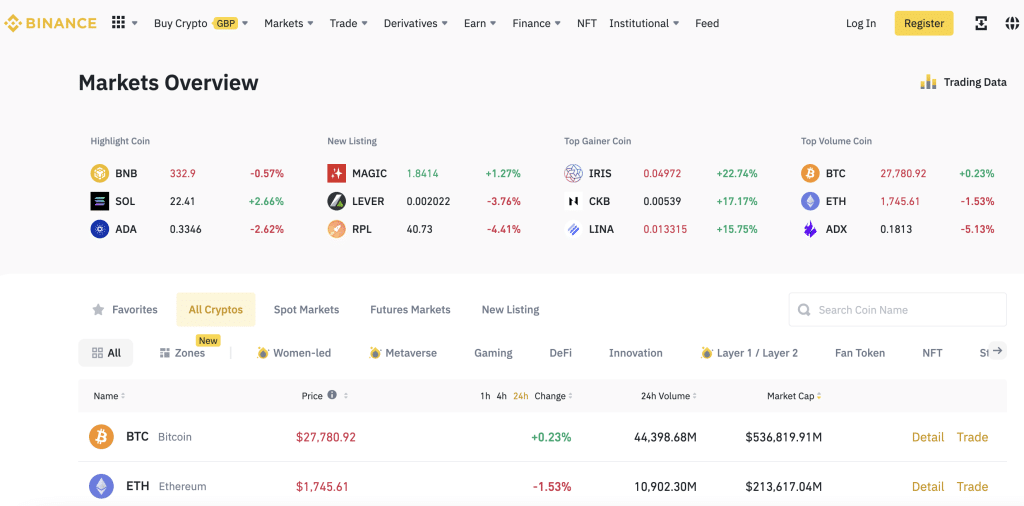This is a detailed screenshot from the Binance website, featuring a white background with a gold-accented top header. In the upper left corner, the word "BINANCE" is prominently displayed in gold capital letters, accompanied by the Binance logo, which consists of two interlocking triangles forming a diamond shape, with three smaller diamond shapes within it. 

The top menu extends from left to right and includes options such as "Buy Crypto" (displaying the currency as GBP for British Pounds), "Markets," "Trade," "Derivatives," "Earn," "Finance," "NFT," "Institutional," and "Feed." On the upper right-hand side, there is a login option along with a gold rectangle button labeled "Register."

Below the header, the main section of the website showcases a headline on the left side that says "Markets Overview." This section lists various cryptocurrencies with associated logos, current prices, and percentage changes indicating whether their value has increased or decreased. The display is organized into four columns, each featuring three cryptocurrencies, including well-known names like Binance Coin (BNB), Ethereum (ETH), and Solana (SOL), among others.

Further down, there is another chart specifically highlighting Bitcoin (BTC) and Ethereum (ETH), detailing their price, percentage change, volume, market cap, and providing options for more details and trading.